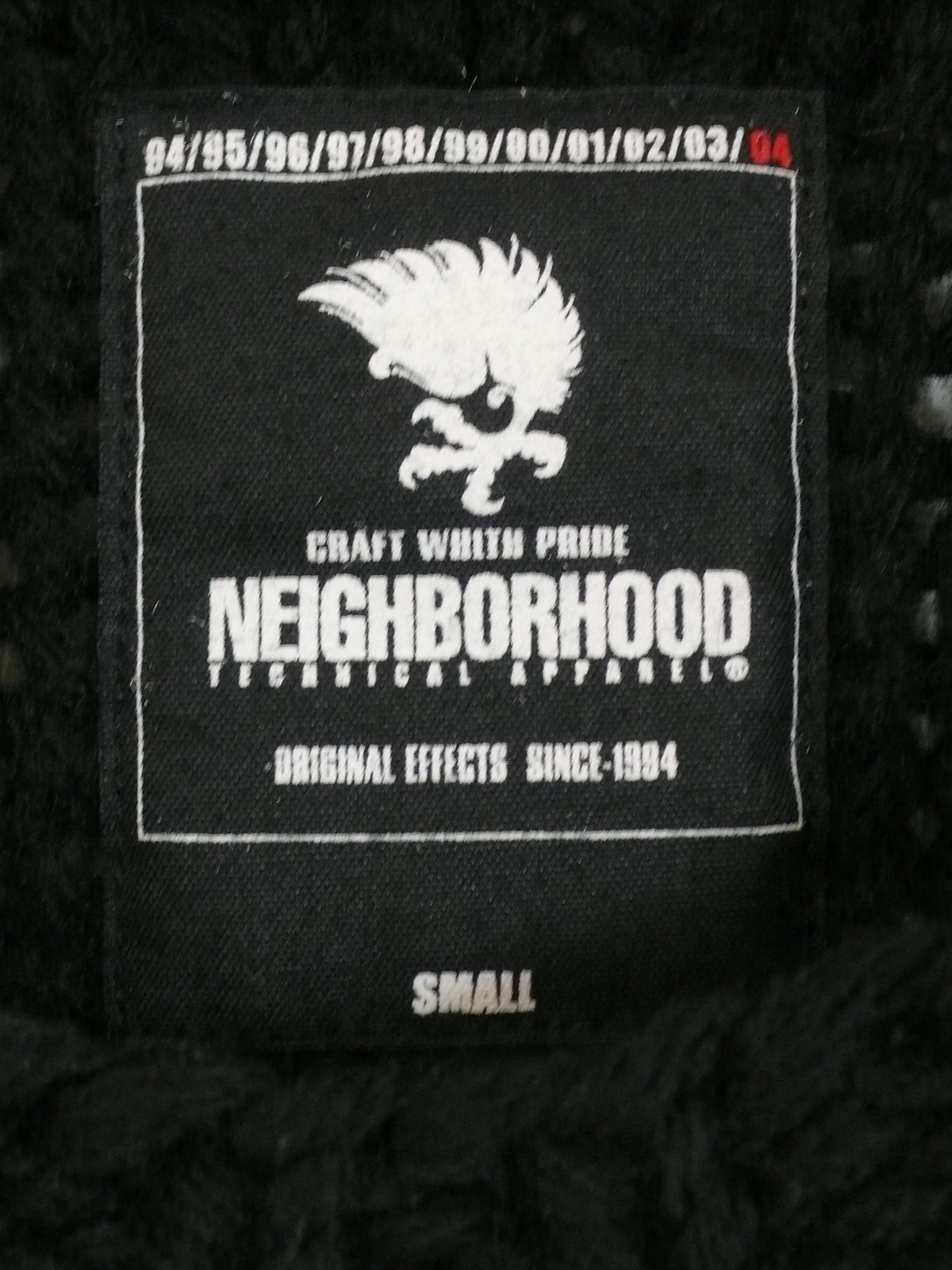This image is a close-up photograph of a black fabric, likely part of a piece of clothing such as a t-shirt, showcasing a detailed design printed in white and red. Dominating the image is a white square outline framing various elements. At the top of the square, a series of years are printed in white text, spanning from '94 through '04, with the '04 highlighted in red. Centrally located is the text "craft with pride" followed by "neighborhood," and "technical apparel," all in white. Additionally, it states "original effects since 1984." Beneath this text is a white bird logo, resembling a hawk, with prominent feathers and a large claw. Outside the white borderline, at the bottom, the size "small" is also displayed in white. The meticulous details and layout suggest both an artistic and informative nature, integral to the identity or branding of the apparel.